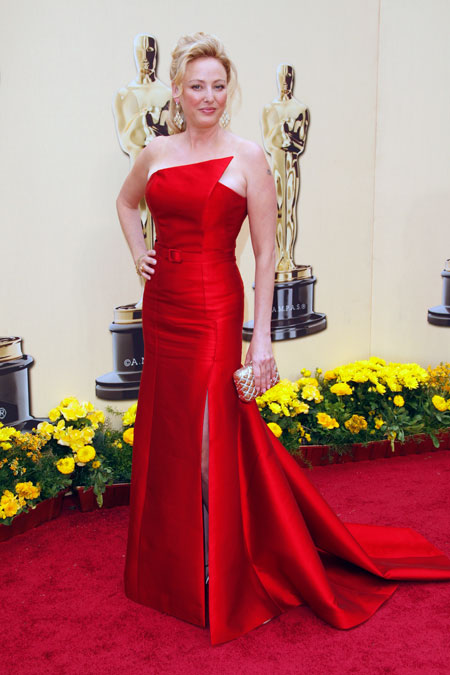The image depicts a white woman, likely a celebrity, standing on a red carpet, possibly at the Oscars. She is adorned in a striking, strapless red gown with a pointed top and a prominent slit on the left leg. The gown is tight-fitting with a medium-sized train trailing behind. Her blonde hair is styled in a wavy updo with tendrils cascading down the left side. She accessorizes with long, drooping earrings that nearly touch her shoulders. In her left hand, she clutches a small, rectangular, gold purse while her right hand is placed confidently on her hip. The backdrop features a cream-colored wall emblazoned with images of Oscars statues on black stands. Bright yellow flowers with green leaves line the ground beneath her, adding a vibrant touch to the scene.